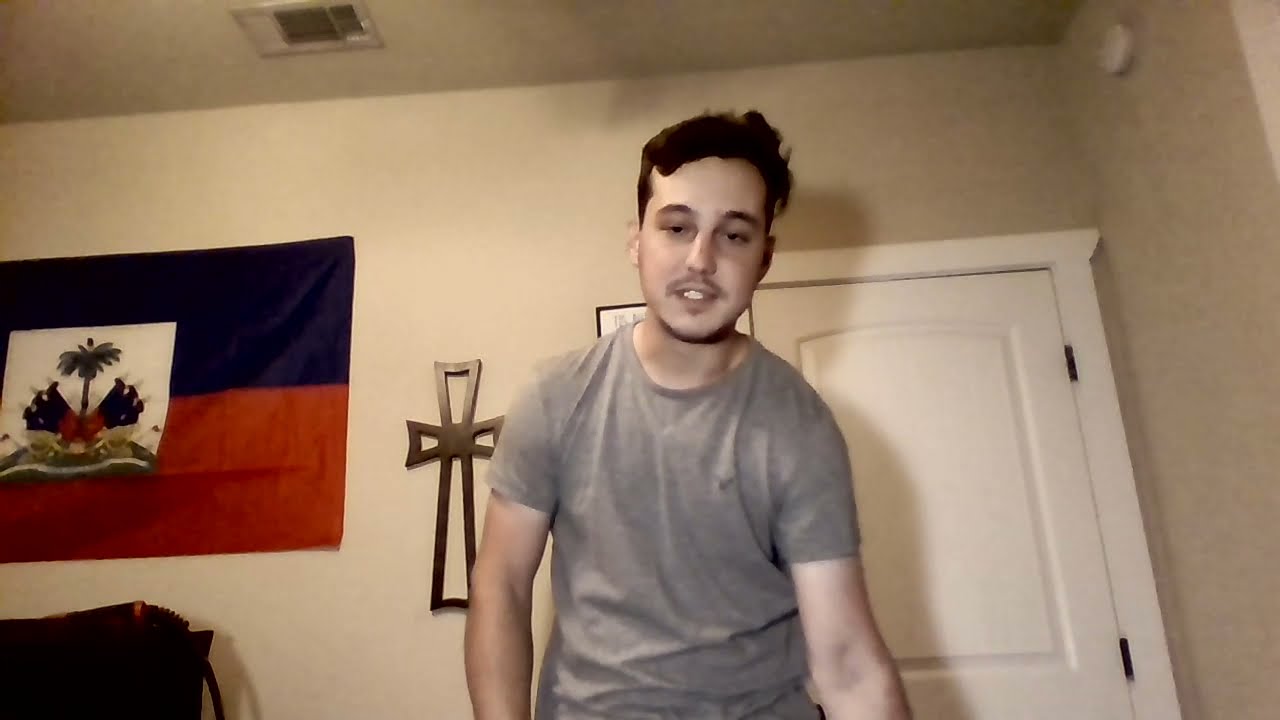The photograph depicts a young Caucasian man with short, unkempt black hair and a slight mustache, wearing a light heather gray short-sleeved t-shirt. The image, taken from a lower angle, captures the man from the hips up, slightly bent over and seemingly engaged in an action such as grabbing, moving, or dancing. He stands in a bedroom with a light beige or brown wall and ceiling visible behind him. Prominent in the background are several key elements: a large white door with white molding and black hinges, a crucifix mounted on the wall, and to the left of the crucifix, a flag divided into blue and red halves with a white square in the center featuring a palm tree and other indistinct elements, possibly a national emblem. Below the flag is a bed, indicating the setting is indeed a bedroom. Additional details include a white smoke detector on one wall and an exhaust vent on the ceiling.